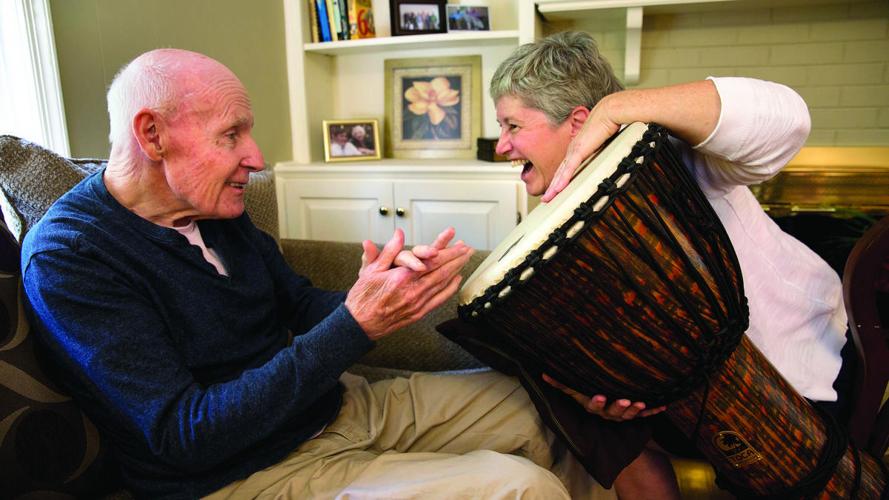In a warmly lit, indoor scene, an elderly couple is captured in a moment of shared joy. The older gentleman, seated in a comfortable recliner on the left side of the horizontally oriented image, wears a blue shirt over a white t-shirt, paired with tan pants. His short gray hair and hands clasped together, fingers intertwined, reflect his excitement and happiness. His gaze is fixed on the woman beside him, who holds a large bongo drum angled towards his knee. She leans forward slightly, her laughter evident as she smiles widely. With short, graying hair, she wears a white top, and her eyes sparkle with mirth as she presents the drum, perhaps reminiscing a fond memory. The bongo, characterized by its brown and black striped base and off-white top, seems to be an object of affection and amusement between them. Behind the couple, a white shelf lines the backdrop, adorned with framed pictures and an assortment of books, further enhancing the cozy, homely atmosphere. This candid, color photograph beautifully captures the essence of companionship and shared happiness in their twilight years.